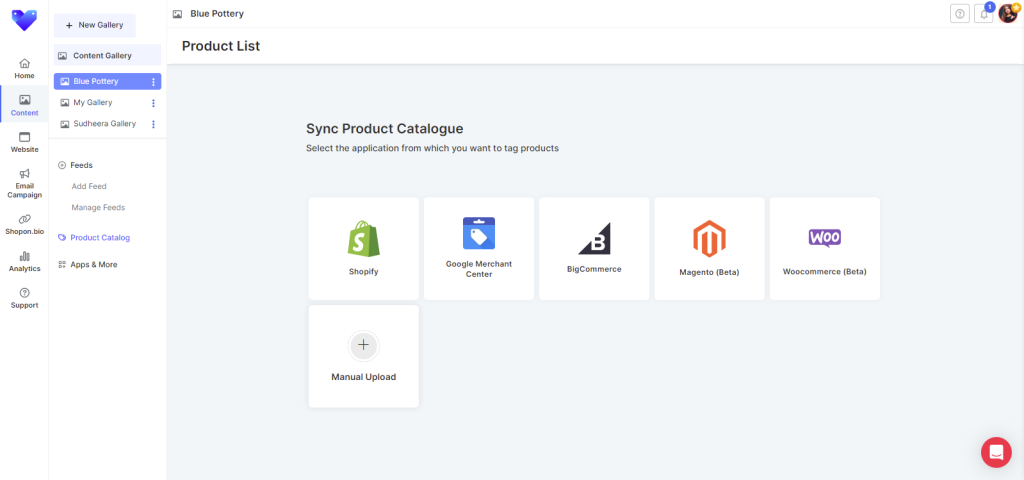The image depicts a webpage titled "Blue Pottery," showcasing a product synchronization system. The layout features a left-hand side menu resembling an email interface, but it is dedicated to navigating different sections of the website. 

Highlighted in the side menu is the section labeled "Content Gallery," under the "New Gallery" category. Other menu options include "My Gallery," "Feeds," "Product Catalog," "Apps," and "More." The far left column displays an icon resembling overlapping shopping tags, symbolizing the marketplace functionality.

The main section of the page shows a list of options to sync product catalogs from various platforms: Shopify (represented by a shopping bag icon with an 'S'), Google Merchant Center, BigCommerce, Magento (in beta), WooCommerce, and a manual upload option.

Additional secondary menu items at the top left include "Home," "Content," "Website," "Support," and "Shopping Info," though the text appears quite small. The overall design and icons use subtle and visually appealing cues to enhance navigation and user engagement throughout the site.